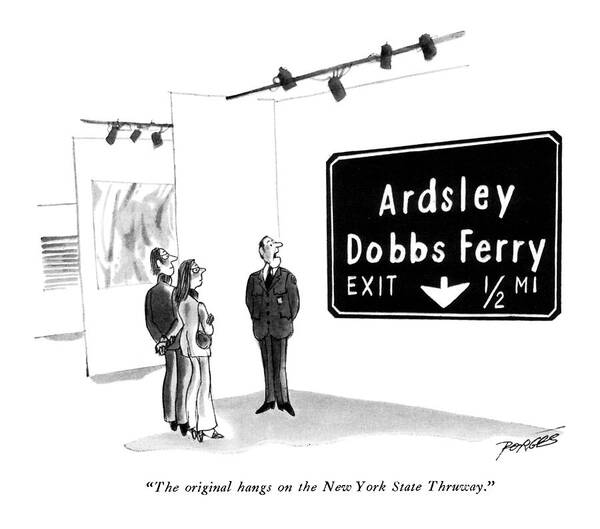This black-and-white comic sketch depicts a scene in an art gallery where three individuals are standing and examining a black signboard illuminated by overhead lights. The signboard, positioned towards the right side of the image, prominently reads "Ardsley-Dobbs Ferry Exit 1 1⁄2 Mile," with an additional note at the bottom stating, "The original hangs on the New York State Thruway." A man in a dark grey suit, presumably a museum curator, is explaining this exhibit to a man and a woman who are examining the sign with great interest. Adjacent to the main exhibit, other less discernible images are visible. The cartoon includes a signature at the bottom right corner, which appears to be "Porges." The overall setting and style reflect typical comic art, emphasizing the humorous juxtaposition of a mundane highway sign within an art gallery context.